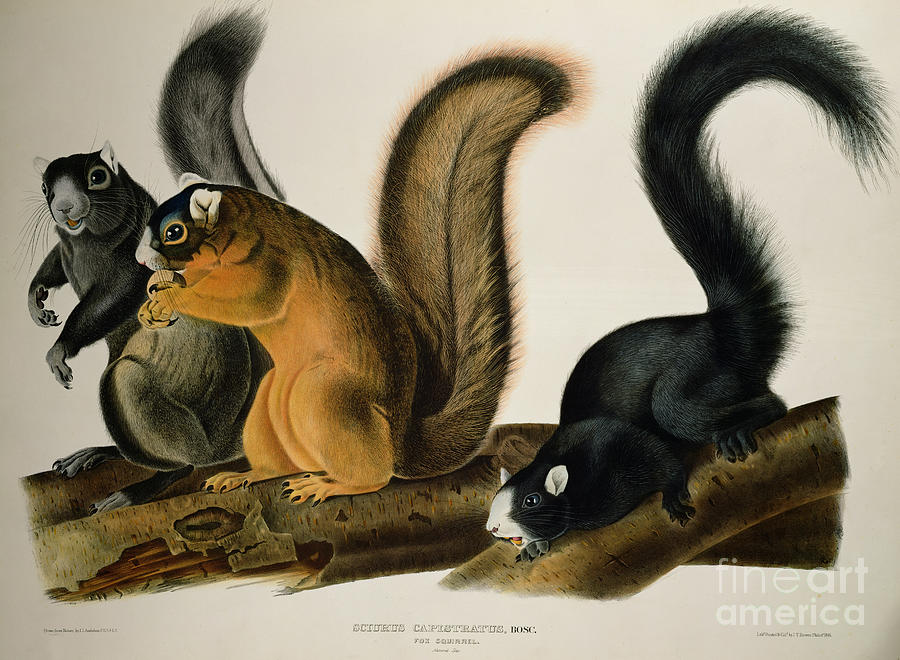This is a detailed, watermarked reproduction of a fine art print reminiscent of John James Audubon's style, possibly attributed to him. The illustration features three distinct squirrels perched on branches that traverse horizontally across the lower portion of the image, with one branch angling slightly to the right. The branches, covered in thin bark akin to cherry or birch, provide a natural setting for the different species of squirrels depicted.

The leftmost squirrel is predominantly black-gray, upright on its haunches, engaging the viewer with a direct gaze. Adjacent to it, the central squirrel is tawny red and is shown in left profile, clenching an acorn between its paws while eating. Both of these squirrels display white ears and upturned tails. The rightmost figure is a younger, entirely black squirrel with a distinct white mark on its nose and chin, white ears, and a long, arching tail that lends it a monkey-like appearance. This squirrel is closer to a horizontal position, firmly clutching the branch with all fours.

Additional details include the artistic watermark "Fine Art America" and indecipherable text beneath the original piece, which likely includes the artist’s name, title, and subject information.